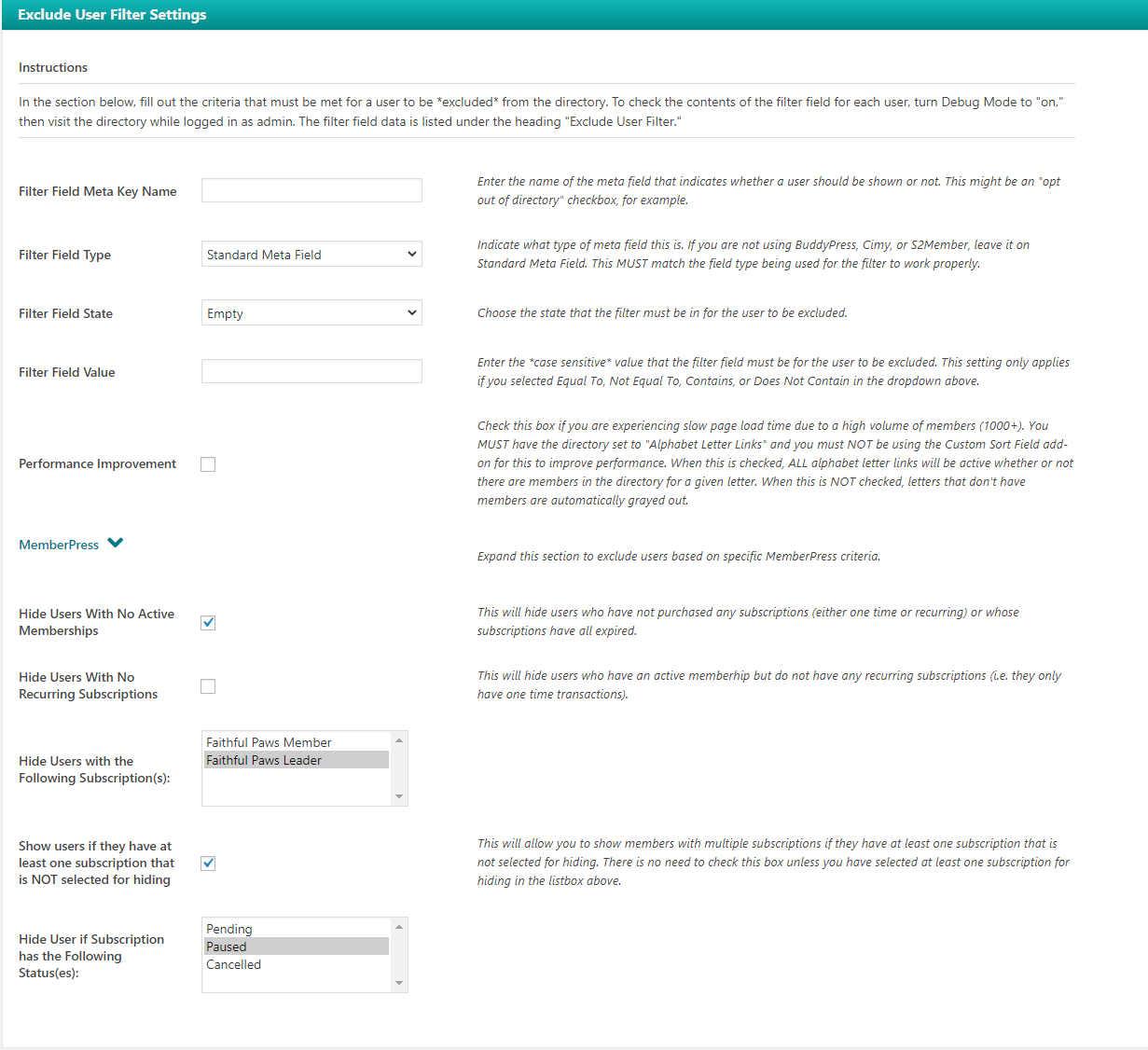### Caption:
The image displays a screenshot of a settings page for an unidentified website or software application. The page is specifically labeled "Exclude User Filter Settings" in the upper left corner. Below the label, there are instructions provided: "In the selection below, fill out the criteria that must be met for a user to be excluded from the directory. To check the contents of the filter field for each user, turn debug mode on, then visit the directory whilst logged in. The filter field data is listed under the heading 'Exclude User Filter.'"

The page includes several fields:
- **Filter Field:** Presumably for specifying the attribute to filter by.
- **Filter Type:** Indicates the type of filter being applied.
- **Filter State:** Possibly denotes the current status of the filter.
- **Filter Value:** The actual value used to determine exclusion.

These settings seem to control the exclusion of users from a directory, possibly to prevent them from accessing, moderating, or editing content on the website. The full context is unclear due to the lack of specific application or platform information.